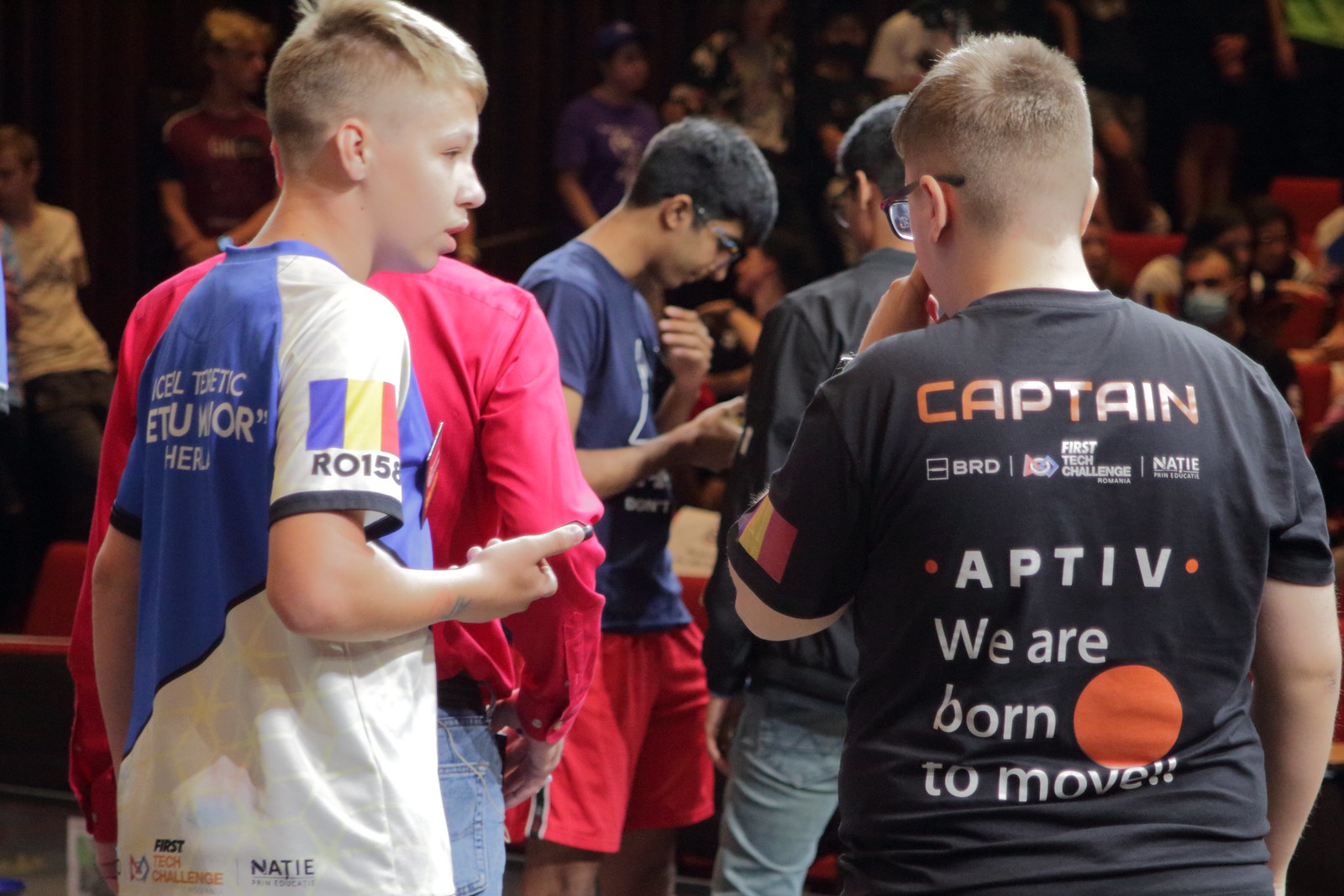This vibrant photograph captures a lively gathering of kids, likely aged around 14 to 16, participating in a competitive event, possibly a sporting or robotics competition. At the center are two prominent young men engaged in conversation. The one on the right, a blonde teenager wearing glasses, sports a black t-shirt with "CAPTAIN" written on the back. This shirt features several logos, including "First Tech Challenge" and "APTIV. We are born to move," with an orange circle above the word 'MOVE.' His shirt also displays a flag with blue, yellow, and red vertical stripes on the sleeve. To his left stands another young man with short blonde hair, dressed in a primarily white t-shirt with blue accents. This shirt mirrors the black one with its flag and has text that reads "RO158" on the sleeve and some logos at the bottom. The two boys are surrounded by other participants and adults. In the distant background, the photo reveals an array of onlookers seated in stands or bleachers, reflecting significant audience interest in the event.